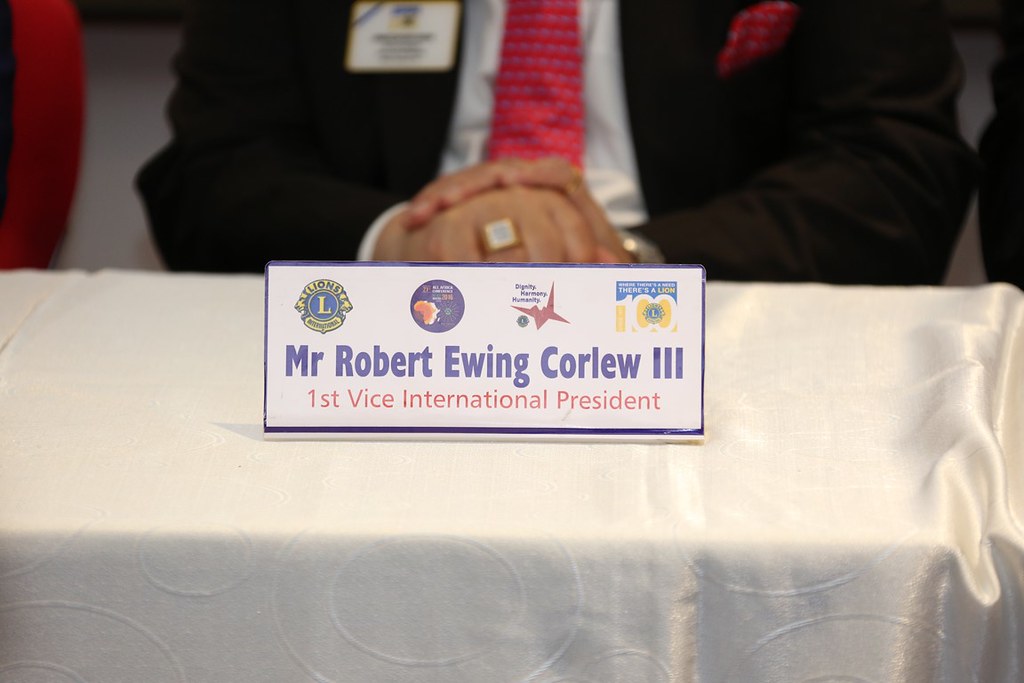This image captures an intense close-up of a nameplate at what appears to be a conference or meeting, focusing on Mr. Robert Ewing Corlew III, who holds the title of First Vice International President. The nameplate, set against a white tablecloth, features a blue border and a white background. Positioned prominently along the upper edge are four colorful logos in various shades of red, blue, and yellow, though their exact details are indistinct. Below the logos, Mr. Corlew's name is written in blue, with his title in red underneath.

Behind the nameplate, the background blurs to reveal the partial image of a man, cut off just below the chest. He is dressed in formal attire, including a black suit jacket with a red pocket square, a white dress shirt, and a red tie. His hands are folded neatly on the table, displaying a square-shaped ring. The backdrop includes hints of additional colors and shapes, suggesting the presence of others nearby, with red to his right and black to his left likely indicating other attendees or furnishings.

The intricate details and the prominent placement of the nameplate emphasize Mr. Corlew's distinguished position at the event, while the blurred background adds a sense of depth and context to the setting.